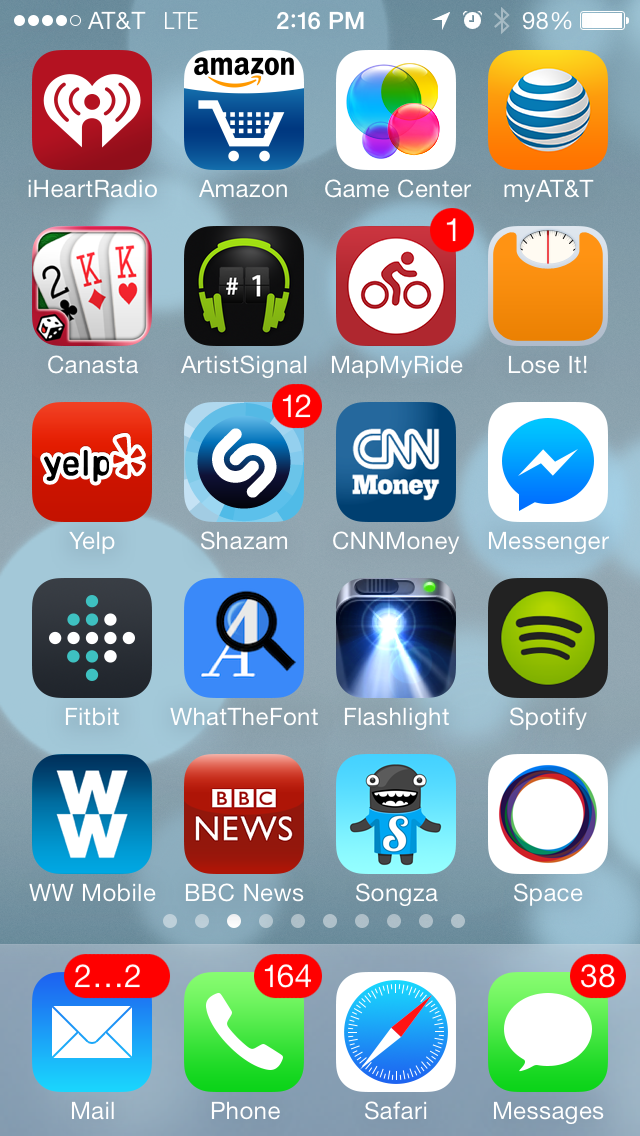This is a detailed description of an iPhone home screen screenshot showcasing a wide variety of app icons. Each app is distinct, illustrated as follows from left to right, top to bottom:

1. **iHeartRadio**: The first app, featuring a red background adorned with a white heart at the center.
2. **Amazon**: A two-tone icon with a blue background displaying a white shopping cart, above which "Amazon" is written in black on a white section with an orange arrow swooping underneath.
3. **Game Center**: Identified by its white background decorated with overlapping blue, yellow, purple, and pink circles.
4. **MyAT&T**: An app with an orange background and a globe with white and blue stripes, representing the brand.
5. **Canasta**: Showcasing playing cards - a two of clubs, a king of diamonds, and a king of hearts.
6. **Artist Signal**: Depicts a black background with green headphones encircling a number one.
7. **Map My Ride**: Displays a red background with a white circle enclosing a red figure riding a bike.
8. **Lose It!**: An orange background resembling a bathroom scale.
9. **Yelp**: Red background with "Yelp" written in black, outlined in white, accompanied by a red and white flower.
10. **Shazam**: Various shades of blue with an 'S' inside a darker blue circle.
11. **CNN Money**: Dark blue background with "CNN Money" in white text.
12. **Messenger**: White background featuring a blue text bubble with a white lightning stripe inside.
13. **Fitbit**: Dark gray background adorned with teal and white polka dots forming a square.
14. **What The Font**: Light blue background with a white 'A' being magnified by a black magnifying glass.
15. **Flashlight**: Black background highlighted by a flashlight beam pointing upwards.
16. **Spotify**: Black background with a green circle and three black swoops across it.
17. **WW Mobile**: Blue gradient background with two stacked white 'WW' letters.
18. **BBC News**: Red background, with "BBC" in white squares and "News" in white text.
19. **Songza**: Pale blue gradient background with a quirky gray figure sporting big eyes and teeth, wearing a blue shirt featuring a big white 'S'.
20. **Space**: White background with a multi-hued, rainbow-colored circle.

At the bottom of the screen, there are essential apps:

- **Mail**: Blue gradient background with a white envelope, showing over 2,000 unread emails.
- **Phone**: Green background with a white phone handle, showing 164 missed calls in a red bubble.
- **Safari**: White background with a blue compass, wherein the hands are half red and half white.
- **Messages**: Green background with a white text bubble, with a red bubble indicating 38 unread messages.

The wallpaper is a grayish-blue hue, interspersed with light blue bubbles floating around. At the top, status indicators show the user is on AT&T's LTE network, the time is 2:16 PM, and the battery is at 98%.